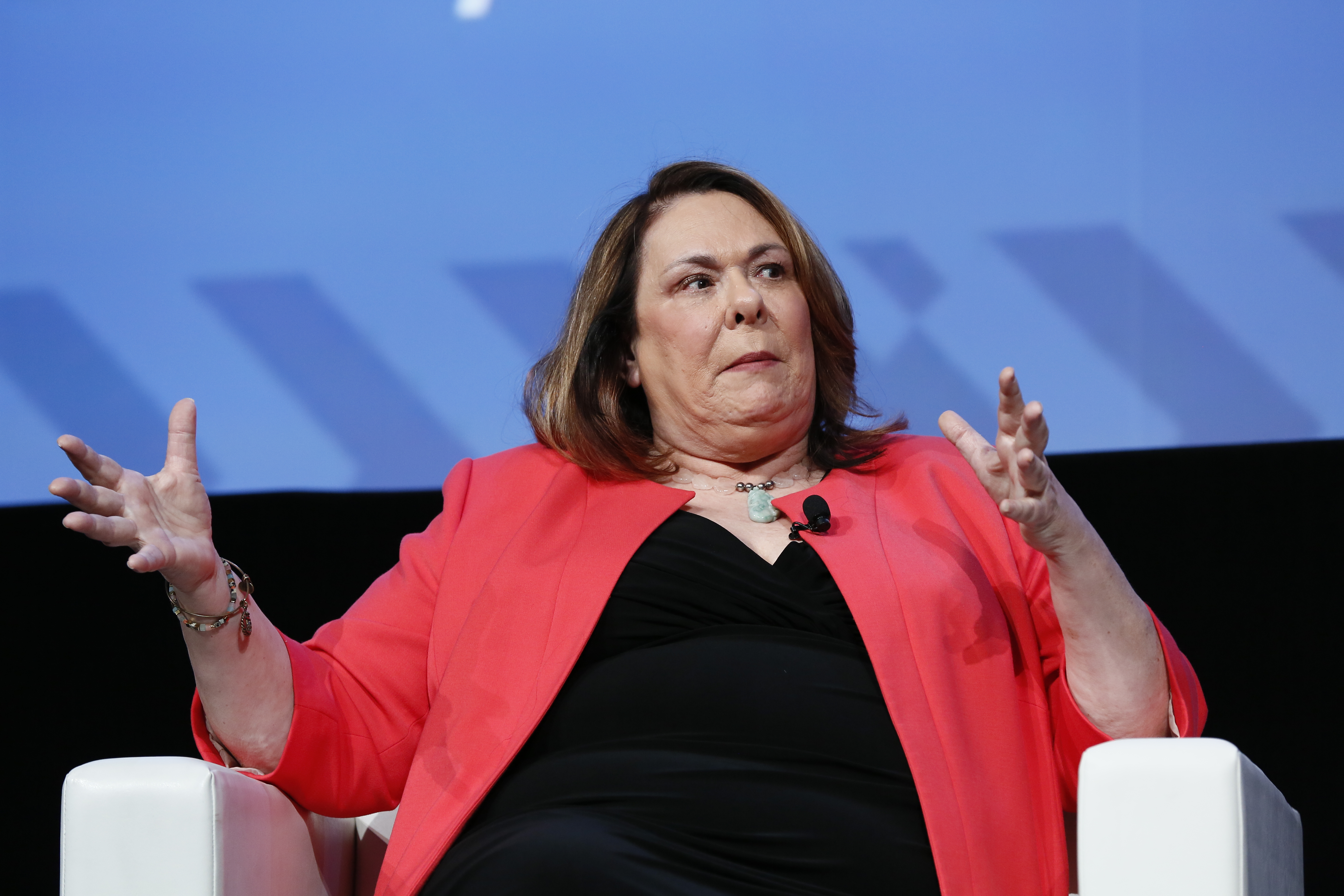The photograph depicts an older woman, likely a politician or spokesperson, seated in a large, solid white chair characterized by its geometric design and right angles. She has a medium haircut with brown hair parted in curtains on either side and wears a red, open-front sweater paired with a black undershirt or dark dress featuring a deep neckline. Her outfit is accessorized with bracelets on her right arm and a necklace with a pale stone pendant. A lapel microphone is clipped to her sweater, indicating she might be speaking publicly. The woman has her arms extended outward, fingers splayed, as if she is expressing concern or vividly describing something. Her expression is neutral, not smiling nor angry, with slightly creased eyebrows. The background features an indistinct design on a blue backdrop, partially out of frame, with a black section cutting off the bottom of the image.